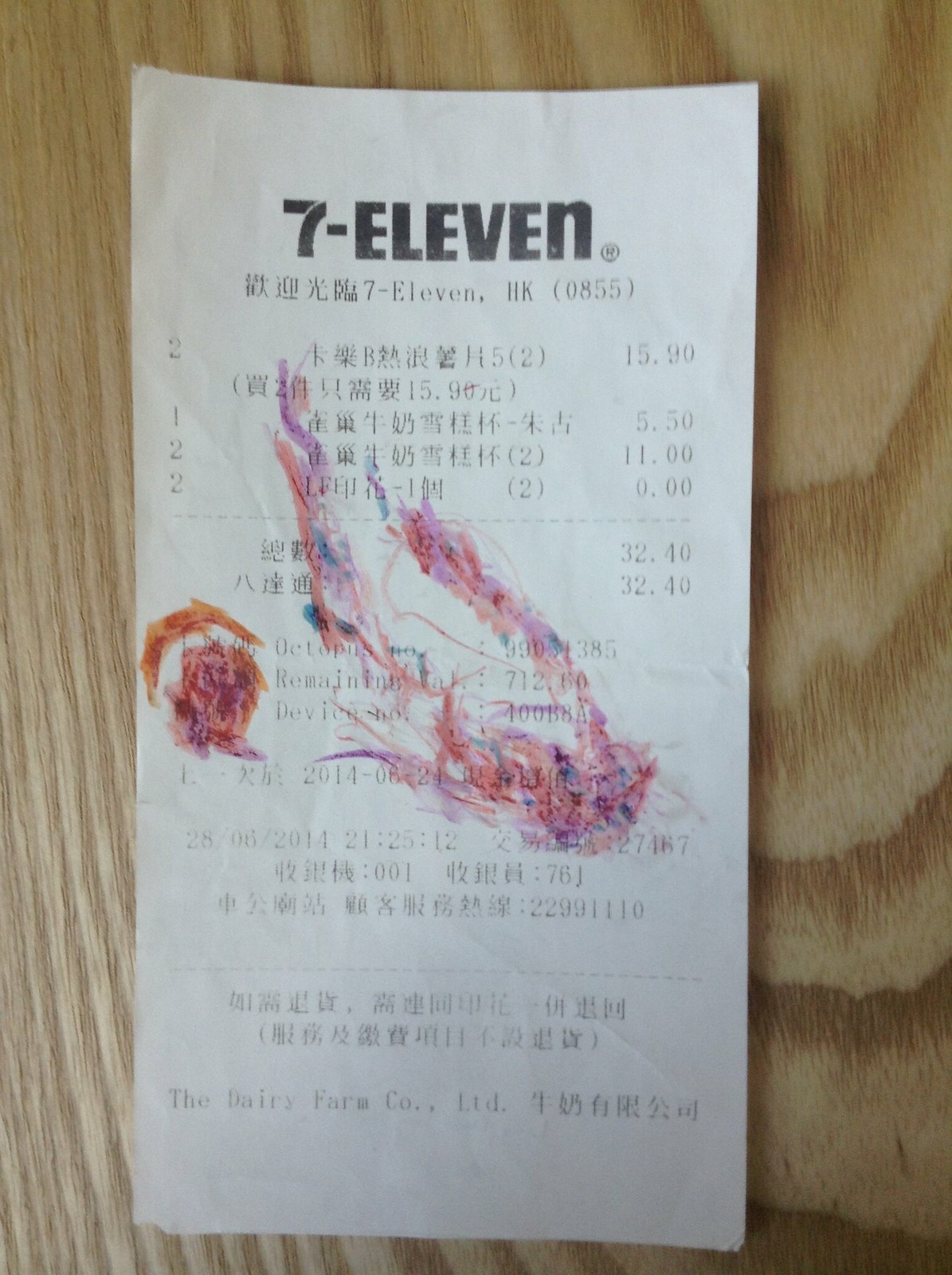A detailed image depicts a small white register receipt lying on a flat, hard wooden surface that showcases an intricate grain pattern. The surface, likely a tabletop, consists of at least two types of light-colored brown wood. Each type of wood contributes a distinct grain pattern; one features nearly vertical lines while the other displays more horizontal rings. 

The receipt clearly reads "7-11" at the top, with the number "7" followed by a dash and "11" spelled out, characteristic of the convenience store chain's logo. Below this, the letters "HK" and the number "(0855)" are visible, potentially indicating the store's specific location. The rest of the characters on the receipt are in an unfamiliar language. 

In addition to the text, the receipt is embellished with an ornate floral design, featuring intricate, multicolored patterns primarily in pink, violet, and blue hues. The design includes two floral objects—a partial ring and a small flower. The combination of the stark white receipt and the rich, natural wood grain provides a visually appealing contrast, further enhanced by the intricate floral artistry on the receipt.